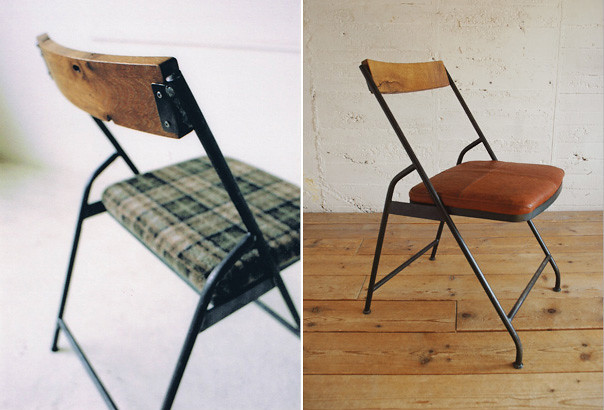This is a detailed photograph consisting of two side-by-side color images showcasing folding chairs with black metal frames, wooden backrests, and cushioned seats. The left image features a three-quarter view of the back of a folding chair placed against an all-white background and floor. The chair has a green and tan plaid cushion for the seat, and a wooden backrest. In the right image, the folding chair is similarly angled but shows the right side, with the cushion facing right. It has the same black metal frame and wooden backrest, but the seat cushion is covered in a tan fabric with an orangish hue. This chair is positioned on an unfinished hardwood floor with a stucco or brick background. Both images emphasize the detailed craftsmanship and differing seat cushions of the chairs, suggesting they are the same chair with different coverings.